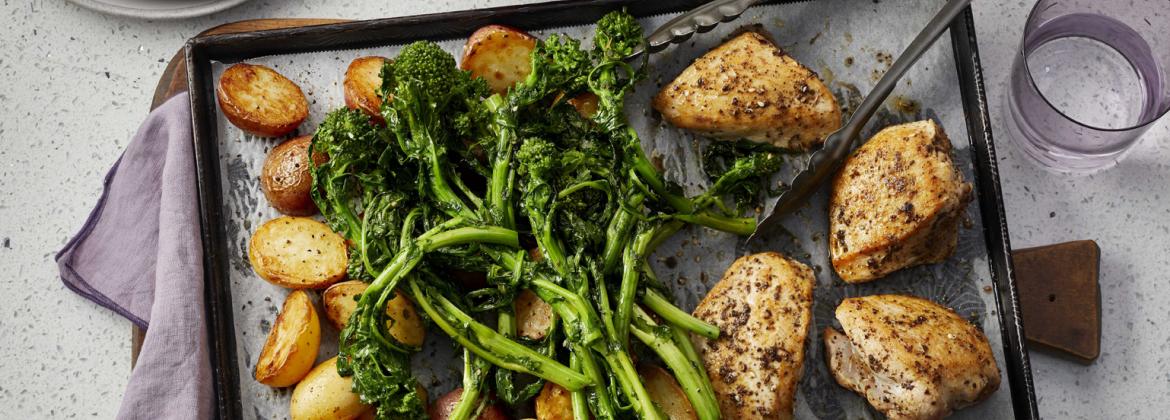This wide, rectangular panoramic image depicts a prepared meal arranged on a black baking tray lined with parchment paper. The left half of the tray features halved baby potatoes, while the right side showcases four large chicken breasts, seasoned with herbs and possibly black pepper. Piled in the center are vibrant green vegetables, likely broccoli rabe or broccolini, with small broccoli-like tips and long asparagus-like stalks. The baking tray rests on a gray tea towel atop a wooden platter, reminiscent of one used for handling pizza, adding a rustic touch. The setting includes a glass of water in the upper right corner and a hint of a white plate on the upper left. The entire scene is set against a speckled cream countertop. Additionally, tongs are positioned nearby for serving the meal.